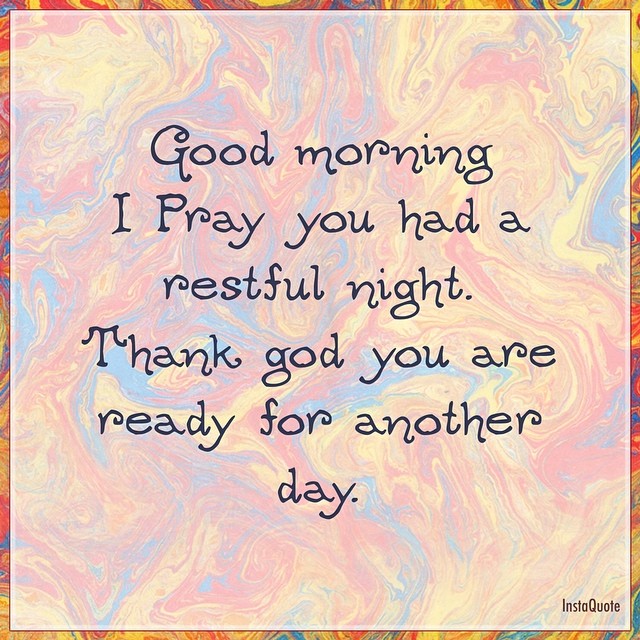**Caption:**

This image features a square sign with a tie-dye marble background in vibrant shades of blue, red, orange, and green. It has a delicate, tiny border encircling it. The background appears very swirly and cloud-like with pastel tones of light blue, light pink, and light yellow, giving it a whimsical, wavy feel. In the center of this background is a heartfelt quote in a black, cursive font that reads, "Good Morning, I Pray you had a restful night thank God you are ready for another day." The words "Pray" are capitalized, and "God" is in lowercase, with "restful night" positioned centrally in a small size to create an appealing, shaped layout. The bottom right corner of the image features the word "InstaQuote" in the same black cursive font, adding an elegant touch to the overall design.